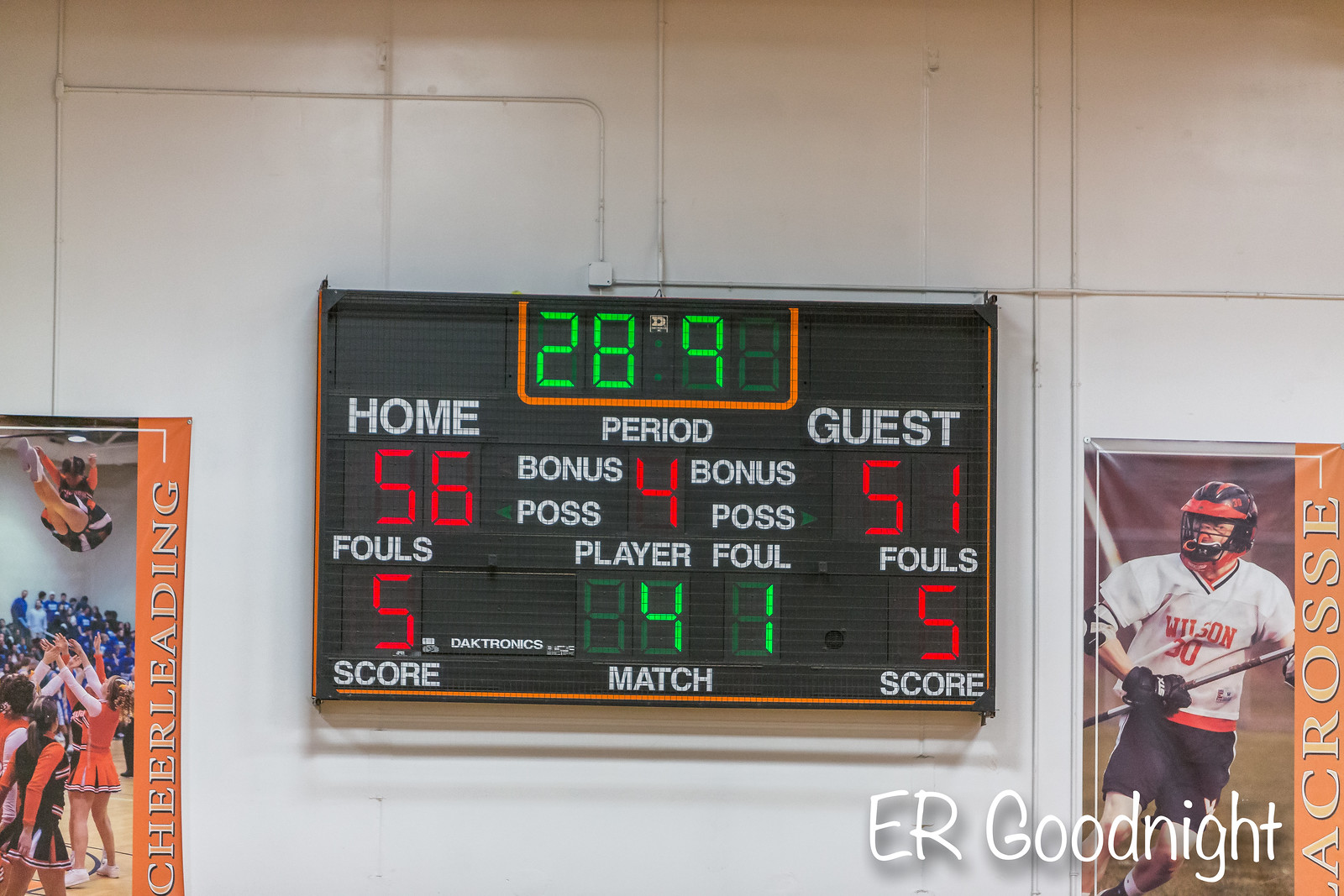This image is a high-resolution photograph taken inside a gymnasium, with the main focus being a large, black digital scoreboard centrally placed against an off-white stadium wall adorned with visible wiring and conduit. The scoreboard displays multiple details: at the top, in green digital numerals, it reads 28-9. The sections below show "Home" with a score of 56 in red, "Guest" scoring 51 in red, the period is indicated as "4" in red, and fouls for both teams are marked as "5" in red. Additionally, “Player fouled: 4-1” is displayed in green. Flanking the scoreboard on either side are two banners with orange stripes. The left banner reads "Cheerleading" and features a photograph of cheerleaders performing a stunt with a stadium backdrop. The right banner, labeled "Lacrosse," depicts a lacrosse player in action with orange, black, and white hues. A watermark in white text at the corner of the image reads "E.R. Goodnight."